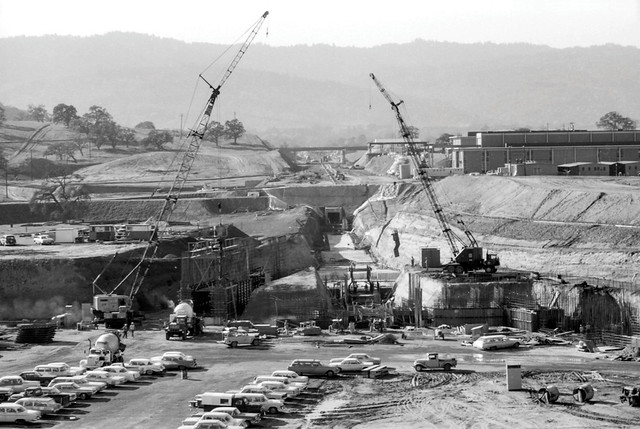This detailed black-and-white photograph from the mid-20th century captures a bustling construction site filled with diverse machinery and vintage vehicles. Dominating the scene are two cranes—one larger crane grounded, and a smaller, shorter-armed crane positioned on an elevated piece of land—possibly engaged in laying down infrastructure such as a tunnel, given the prominently dug ditch. The foreground showcases a sprawling parking lot packed with dozens of cars, likely from the late 1940s to early 1950s, probably belonging to the construction workers. Scattered across the site are various pieces of heavy machinery, including a cement truck with its distinctive barrel, and rebar standing upright, indicating ongoing foundational work. To the left, there's a discernible row of cars atop a hill alongside mounds of dirt and partially dug-out sections of the ground. A tree line and several hills frame the background, with an overpass road faintly visible in the distance. Near the construction, there is a finished two-story building resembling a warehouse and another structure, possibly a school, with windows. This historical snapshot vividly documents the scale and industrial activity of a large-scale mid-20th-century construction project against a backdrop of natural terrain and early automotive history.